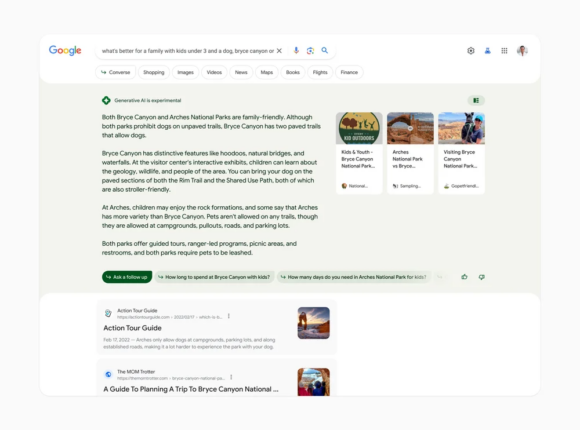An individual is seen using Google to search for information suitable for a family with children under the age of three and a dog, specifically comparing Bryce Canyon and Arches National Parks. The on-screen text is small, but the results prominently feature suggestions powered by Google’s version of generative AI, referred to as "Claude." The AI-generated suggestions inform the user that both Bryce Canyon and Arches National Parks are family-friendly destinations. The description highlights that children might particularly enjoy the rock formations at Arches National Park. Below the AI suggestions, there are additional links, including an "Action Tour Guide" and a "Guide to Planning a Trip to Bryce Canyon." The AI section also includes three related articles providing further details about visiting either Bryce Canyon or Arches National Parks.